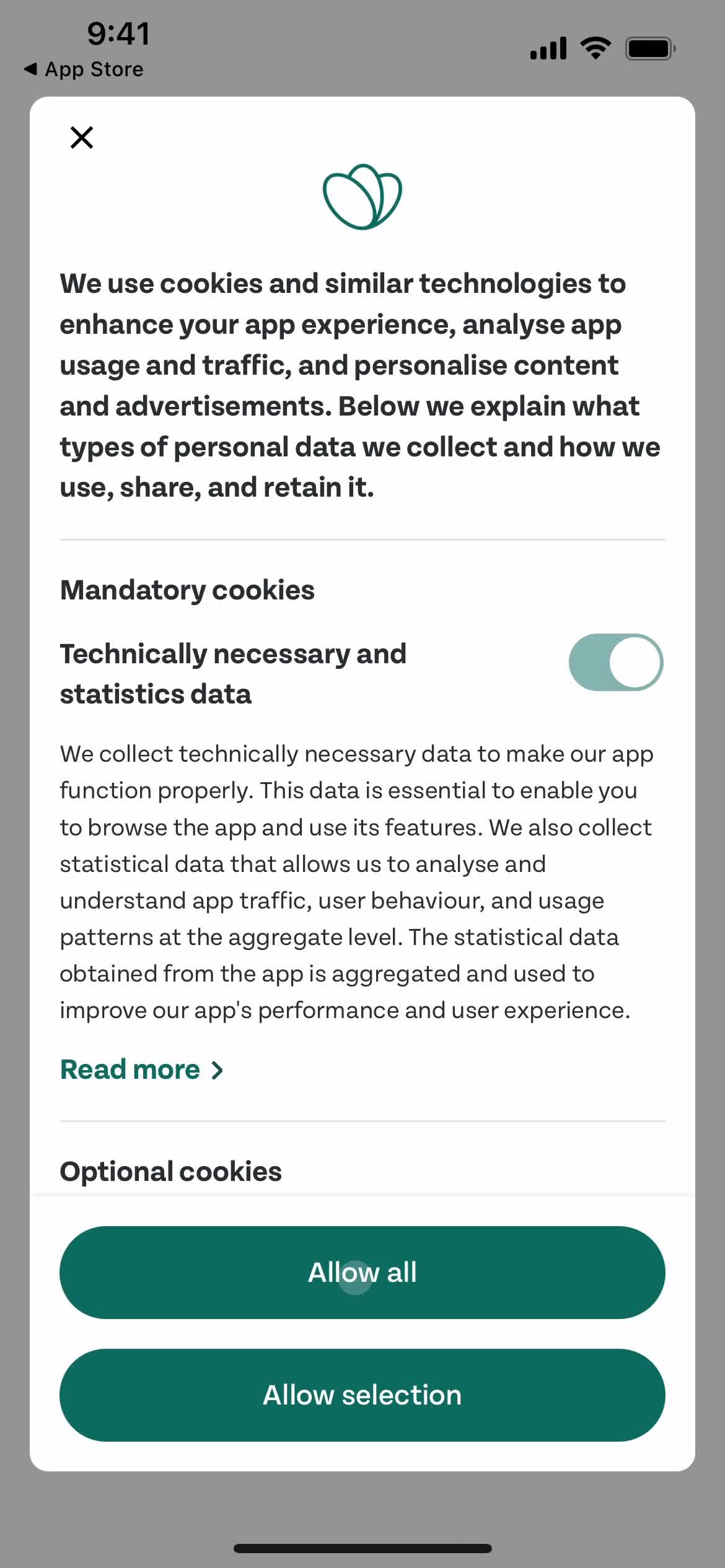A detailed screen capture of a smartphone display at 9:41 AM with a fully charged battery and excellent signal, Bluetooth, and antenna strength indicators. The screen features a notification stating, "We use cookies and similar technologies to enhance your app experience, analyze app usage and traffic, and personalize content and advertisements. Below, we explain what types of personal data we collect and how we use, share, and retain it."

Next, a section titled "Mandatory Cookies" is noted, with a slider set to 'On,' indicating that these cannot be turned off. The description clarifies that technically necessary data is collected to ensure the app functions properly. This essential data allows users to browse the app and utilize its features. Additionally, statistical data is collected to analyze and understand app traffic and user behavior patterns in aggregate form, aimed at improving the app's performance and user experience.

Options for "Optional Cookies" follow at the bottom of the screen, with choices labeled "Allow All" and "Allow Selection."